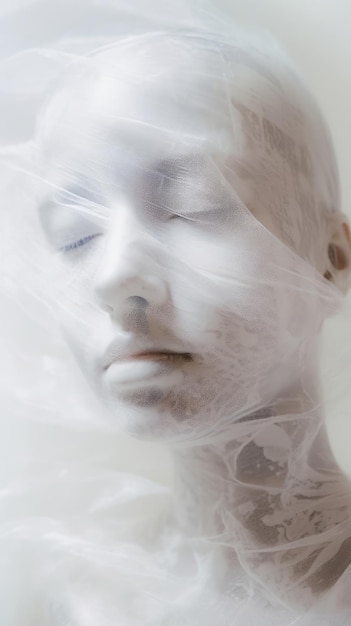This digital portrait, possibly AI-generated, captures the serene and enigmatic visage of a human subject whose gender is indeterminate. The headshot focuses on the face and neck, both shrouded in a gauzy, semi-transparent white fabric that imparts a surreal, underwater or cloud-like quality to the image. The subject appears bald, with closed eyes reflecting tranquility, and their skin exhibits an almost translucent whiteness. The photograph prominently features the left ear, while the right ear remains obscured. The gauzy material, resembling a veil or webbing, drapes elegantly over the top of the head and face, extending into the air to the left of the subject and encircling the neck area, where varying shadows create a slightly darker contrast. The image, predominantly white and ethereal, stands out for its dreamlike and otherworldly atmosphere.